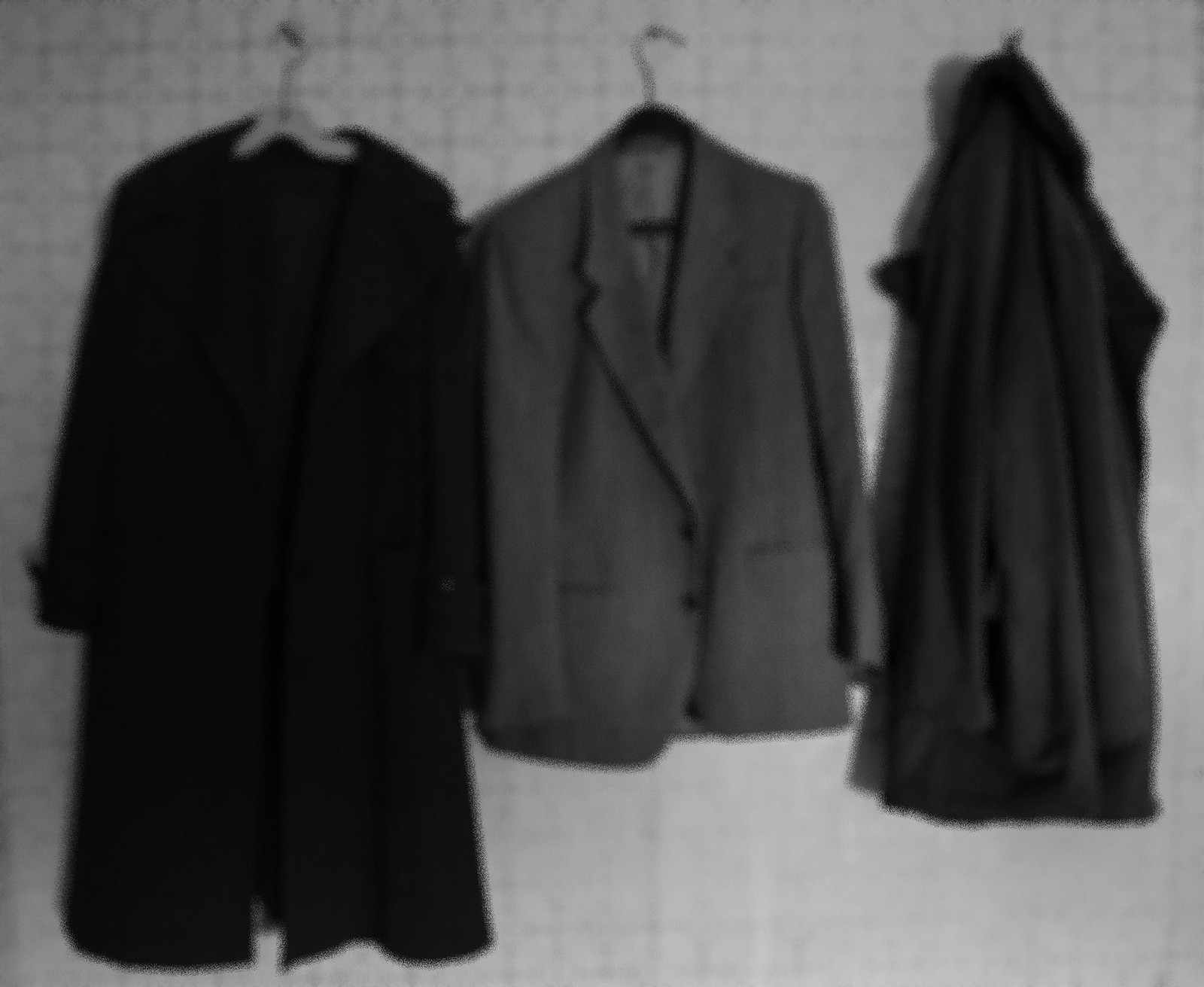This black and white image captures three coats hanging on a wall, presenting a straight-on view. The wall itself has a grid-like pattern, which might be patterned wallpaper or tiles, giving a gray and white appearance. The coats are fixed on large nails hammered into the wall. 

The first coat on the left is black and appears to be a long overcoat with a wide collar that spreads to the shoulders and opens down the front, likely ending just around the knees or slightly lower. It's hung on a white plastic hanger with a metal hook. 

The middle coat is a gray blazer, possibly made of tweed, hung on a black plastic hanger with a right-facing metal hook. 

The third coat on the right is dark gray and notably shorter, possibly waist-length. Unlike the others, it is not hung on a hanger; instead, it is draped directly on the nail using the loop at the back of its neck.